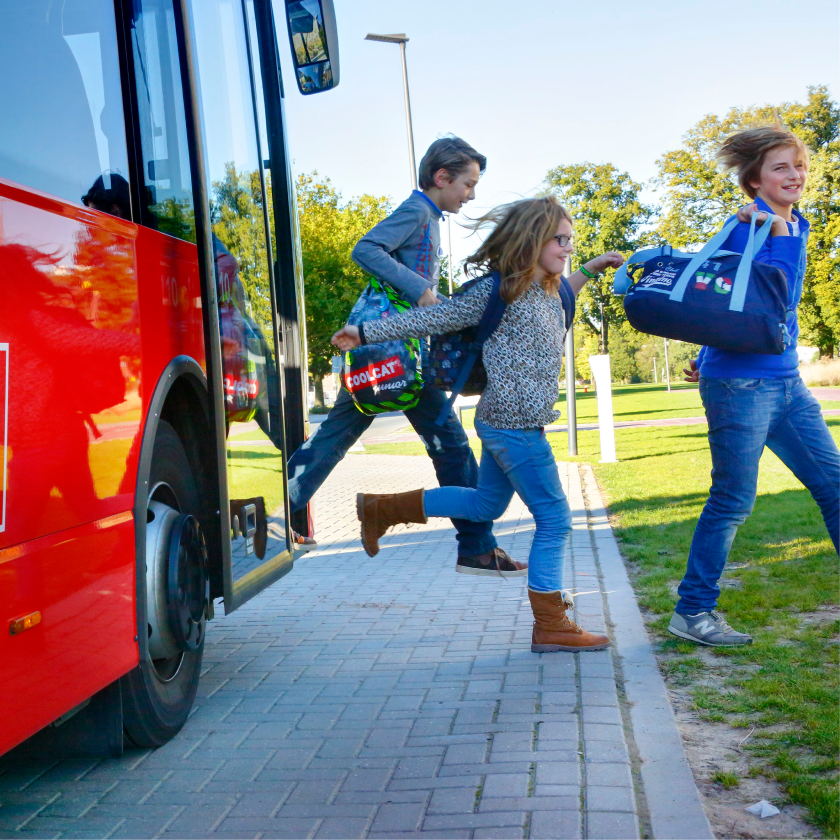The image captures a vibrant moment as three children leap off a bright red bus, which has its fully open sliding door revealing a cobblestone sidewalk and patches of green grass. Leading the group is a young blonde boy, around 12 or 13 years old, carrying a blue duffel bag adorned with Italian flag colors and the letters "VG." He is dressed in a royal blue long-sleeved shirt, blue jeans, and gray New Balance sneakers. His short, blonde hair frames his eager face as he jumps onto the cobblestones.

Following closely is a blonde girl with shoulder-length hair. She sports dark-framed glasses and is energetically skipping off the bus. Her outfit includes a black and gray cheetah print top, blue jeans, and brown lace-up boots. A navy blue backpack sits snugly on her shoulders, complemented by a green bracelet on her wrist. 

The last child, another blonde boy also around 12 or 13 years old, has short hair and is wearing a gray long-sleeved shirt, blue jeans, and brown tennis shoes. He carries a gray bag with lime green and black stripes, prominently displaying a red emblem that reads "Cool Cat."

The bus they are alighting from features a detailed exterior with a red body, black trim around the wheel wells, and visible metallic rims with plastic black outer covers. The lively scene is illuminated by bright and sunny weather, capturing the children mid-leap onto the cobblestone path, ready to explore their surroundings.